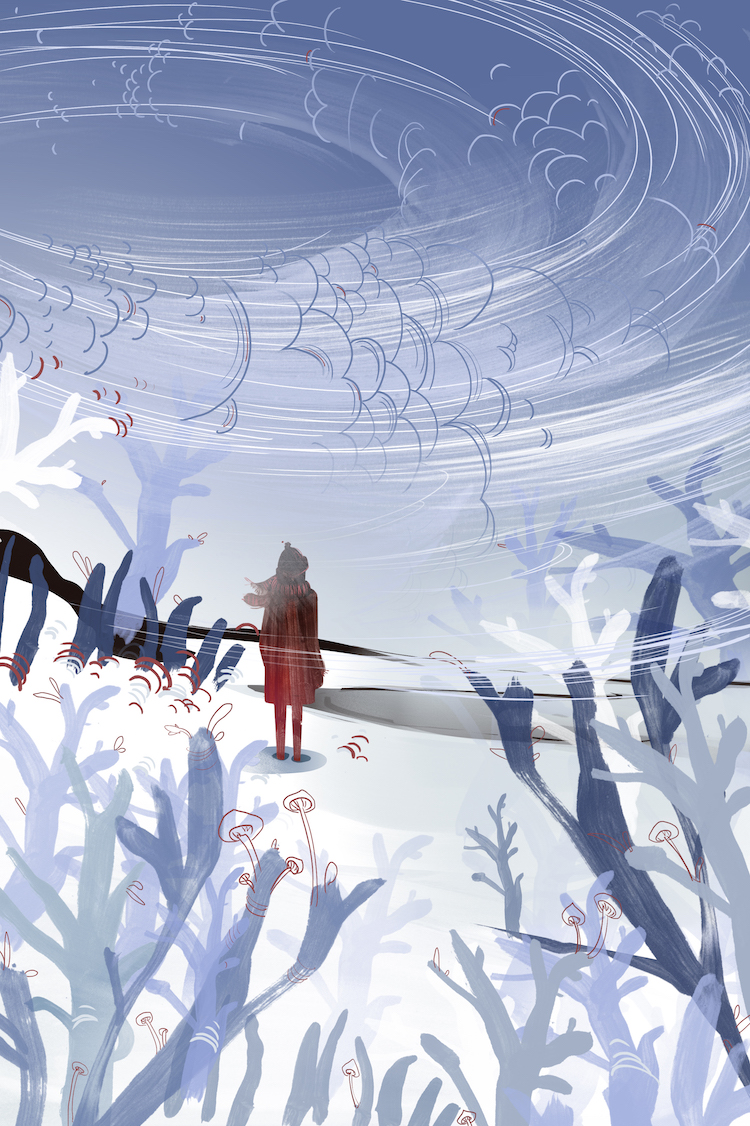The image is a whimsical, anime-style drawing set in a snowy, mystical winter wonderland. Dominating the scene is a figure, likely a young girl, dressed entirely in red—a coat paired with matching pants or stockings and black shoes. She stands still in the snow, facing away from the viewer, gazing into the distance towards the right. Surrounding her are varied shades of blue trees and abstract plant forms, some with red, mushroom-shaped flowers or petals. The backdrop and sky are filled with swirling white patterns that suggest a gusting wind, creating a sense of motion and adding to the enchanting, otherworldly atmosphere of the scene.